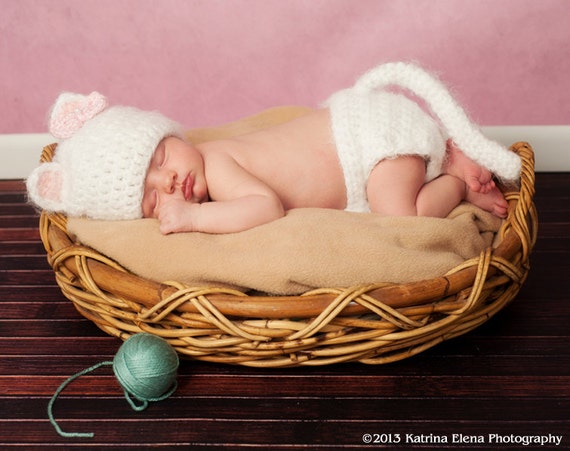This professional photograph, taken by Katrina Elena in 2013, features a tiny infant peacefully sleeping in a woven basket positioned centrally on a soft tan blanket. The baby is adorned in a knitted white cap with two pink ears and matching white shorts with a playful tail. The serene setting includes a dark mahogany-colored wooden floor with horizontal slats, adding rustic charm, and a backdrop of a pink wall with a white baseboard. A silvery blue ball of yarn rests beside the basket on the left, complementing the scene’s cozy, handmade aesthetic.